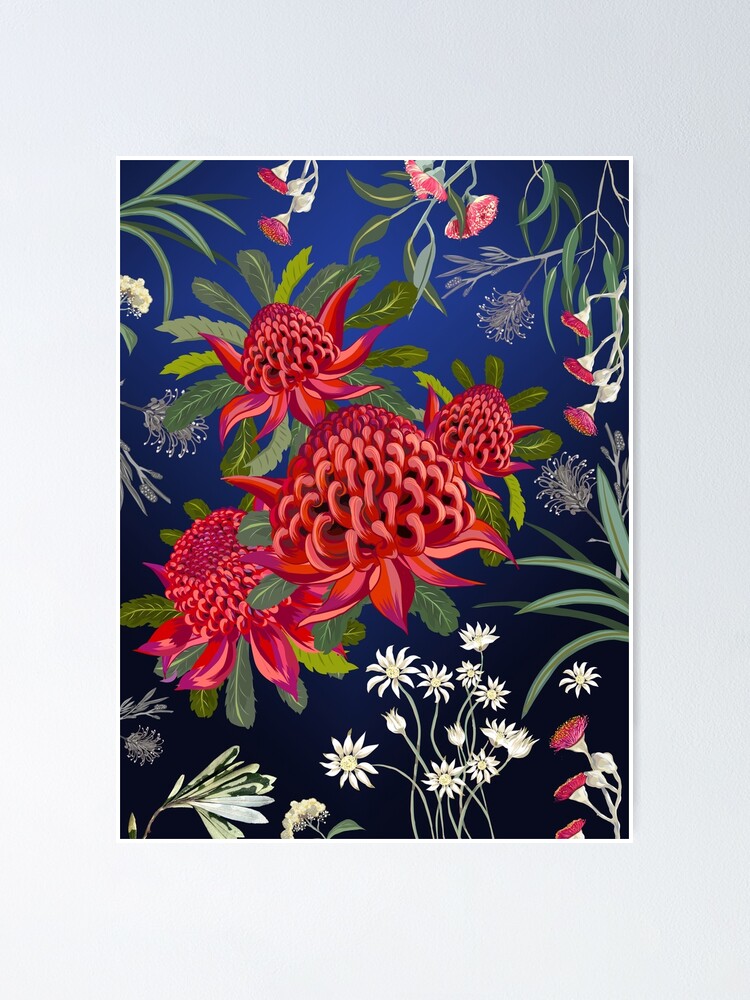This framed piece of modern art depicts a vibrant and detailed floral arrangement against a gradient blue-to-black background. At the forefront are four large, bright red flowers resembling animated strawberries or raspberries, each adorned with ornate green leaves. The bottom center showcases white, daisy-like flowers with delicate stems, while in the low right corner, pink thistle-like flowers grow on white stems. Additionally, the upper right corner features strands of flowers with hanging red cups, and throughout the piece, various flowers dangle like trumpets or resemble fluffy dandelion seeds. All these elements are set off by a light gray frame and a subtle white mat, enhancing the painterly quality of this floral composition.